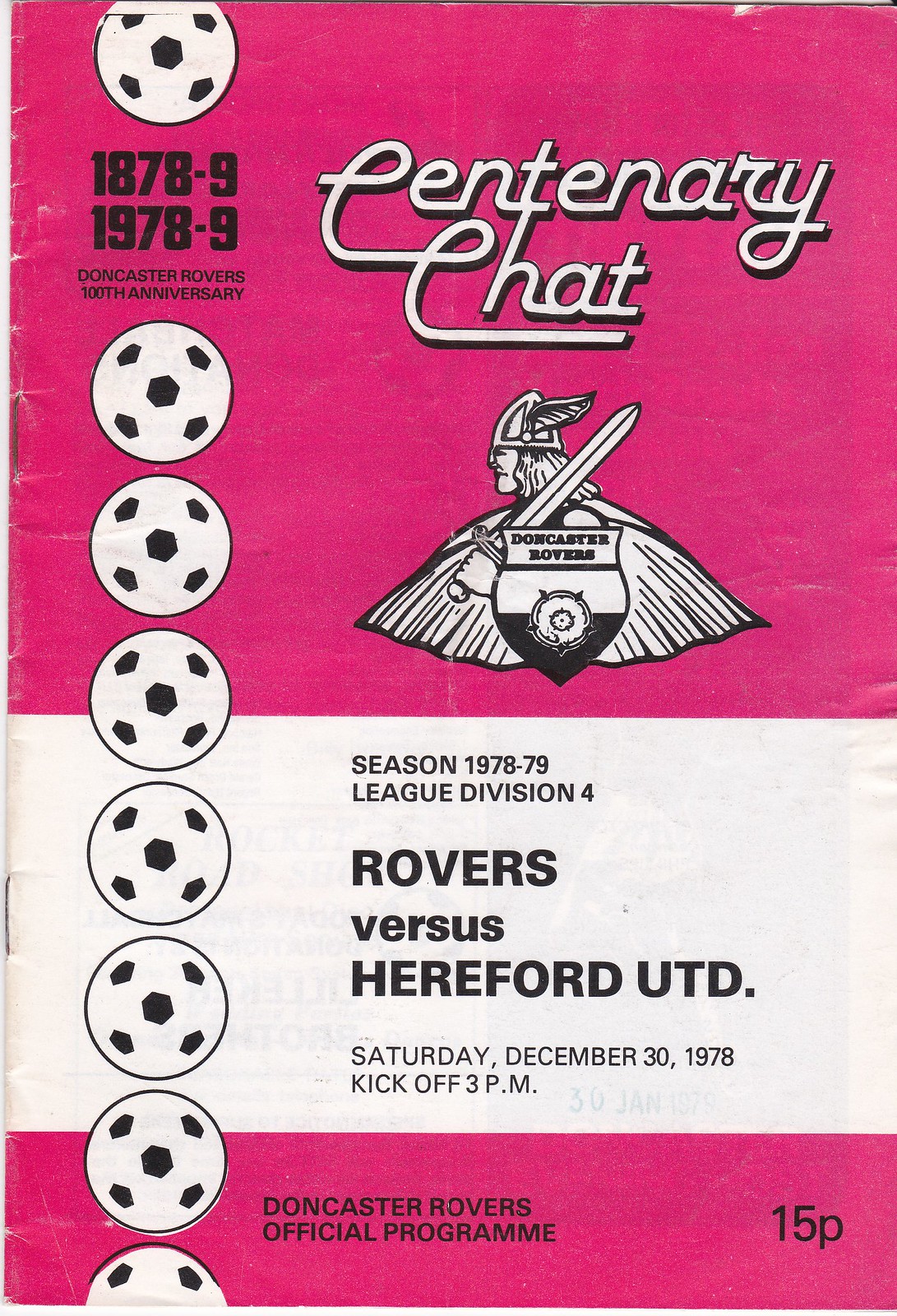The image depicts an official program poster for the Doncaster Rovers' 100th Anniversary, characterized by a distinctive color scheme of pink and white. The layout consists of three horizontal sections with the top and bottom in pink and the middle in white. Running vertically down the left side is a column of soccer balls. Between the topmost soccer balls, it reads "1879-9" and "1978-9" in small lettering, framing the text "Doncaster Rovers 100th Anniversary."

Prominently featured at the center top is the title "Centenary Chat" in white letters. Below this title is an emblematic Viking figure wielding a sword, adorned with a winged helmet. The Viking holds a shield inscribed with "Doncaster Rovers," bearing a divided black and white design. Further detailing the program, it states "Season of 1978-79, League Division 4" against the white background. Below that, crucial match details are noted in small black letters: "Rovers versus Hereford UTD, Saturday, December 30th, 1978, kickoff 3pm." Finally, at the bottom of the pink section, it confirms "Doncaster Rovers Official Program, 15 pence."